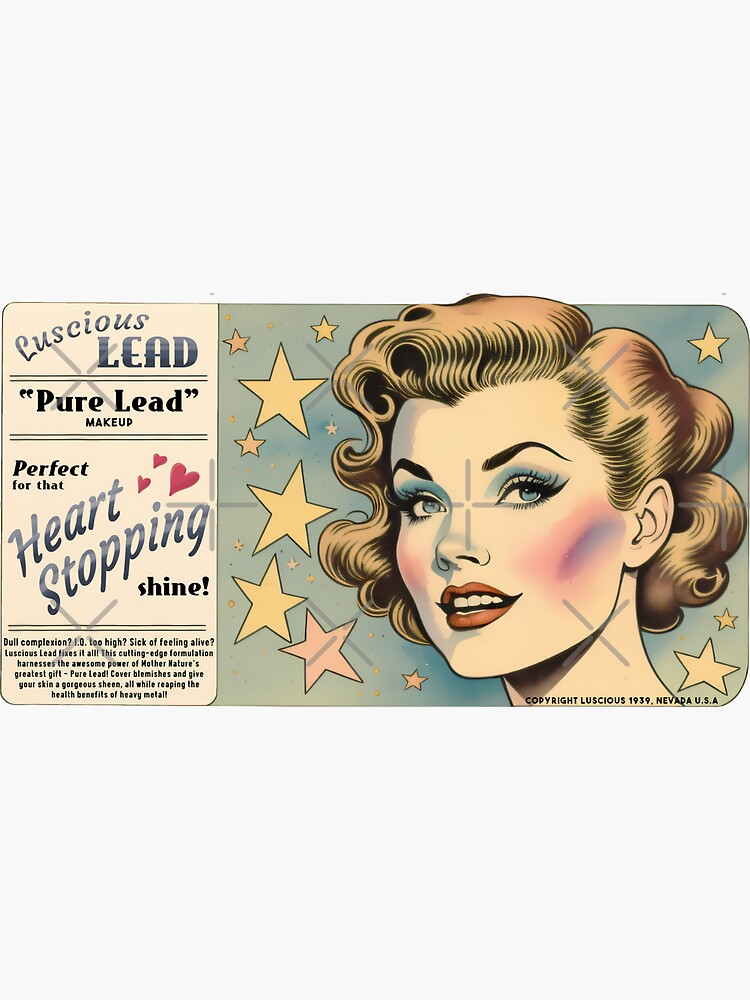This vintage-style advertisement from 1939, illustrated with a light blue hue, features a woman with short, old-fashioned curls in light brown, reddish hair. Her pallid face contrasts with exaggerated makeup, including high-arched black eyebrows, blue eyeshadow complementing her blue eyes, and distinctly red lips. Her rosy cheeks sport purple-blue blobs, and she's smiling with an open mouth. The background is dotted with yellow and red stars, creating a whimsical, eye-catching effect. On the left side of the image, within a tan vertical rectangle, blue text boldly proclaims: "Luscious Lead, Pure Lead Makeup. Perfect for that heart-stopping shine. Dull complexion? IQ too high? Sick of feeling alive? Luscious Lead fixes it all. This cutting-edge formulation harnesses the awesome power of Mother Nature's greatest gift—pure lead. Cover blemishes and give your skin a gorgeous sheen, all while reaping the health benefits of heavy metal." At the bottom right corner, the ad is marked with "Copyright Luscious 1939, Nevada, USA," authenticating its vintage appeal.